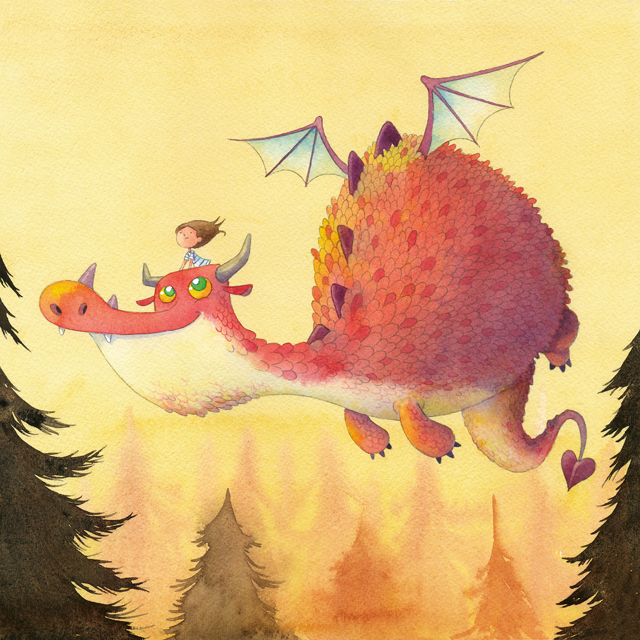A vibrant, cartoon-style image features a large, dragon-like bird soaring through a pale yellow sky. The dragon's body is primarily pinkish-red with darker scales and has a prominent, tall hump on its back adorned with tiny, light blue wings edged in purple. Its underbelly is white. The dragon has green, yellow-accented eyes, purple spikes along its back, and a heart-shaped tail tip. Perched atop its head is a small child with long brown hair, wearing a blue and white striped shirt. The scene is set against a background of watercolor-like evergreen trees that vary—from dark green and yellowish-green on the left, to light brown and orange, fading into the distance. The sides of the image are framed by dark brown, nearly black tree trunks, giving the scene depth and a whimsical quality.